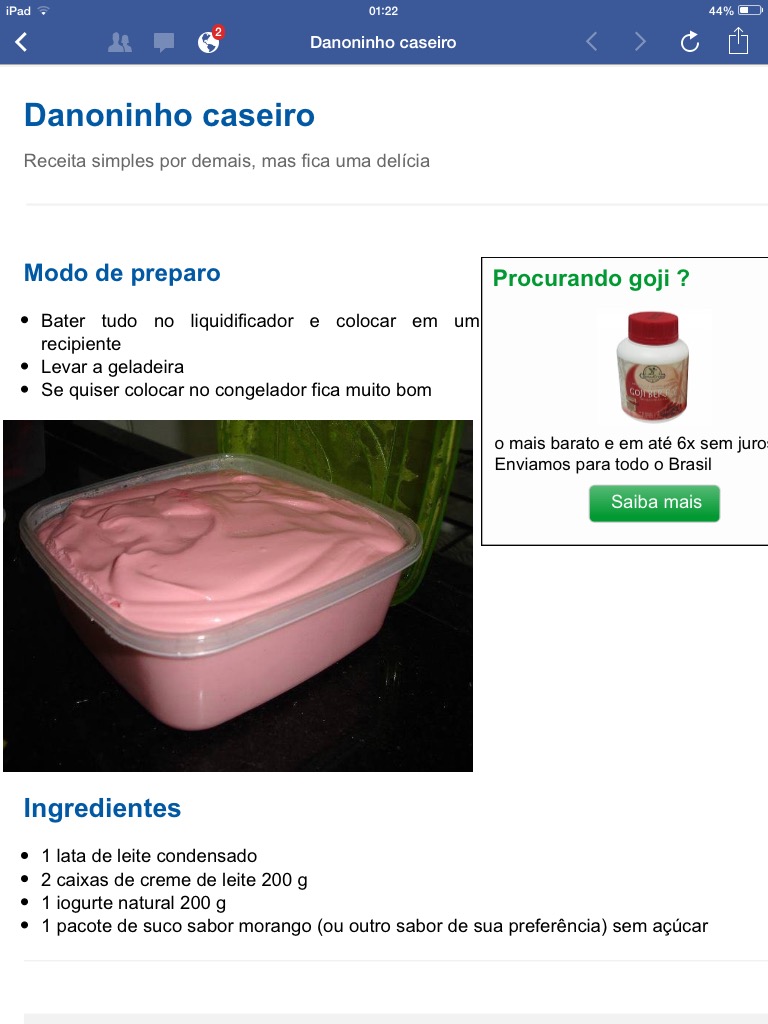This is an image of a screenshot taken on an iPad, which is visible from the "iPad" label in the upper left-hand corner. The picture captures a Tupperware container filled to the brim with a fluffy, pink, pudding-like substance that resembles frosting, icing, or Cool Whip. The Tupperware sits on a black counter, with its lid off to display the contents. The screenshot appears to be of a recipe written in a foreign language, specifically Portuguese.

At the top of the image, the title "Dananinho Caseiro" is displayed in blue ink. Below this, in smaller text, there is another subtitle in blue ink that reads "Modo de Preparo," which translates to "Method of Preparation." This section contains three bullet points with step-by-step directions. Further down, another blue-inked heading says "Ingredientes" or "Ingredients," followed by a list of four bullet points detailing the necessary items: one can of sweetened condensed milk, two packets of cream, one natural yogurt, and one packet of strawberry-flavored juice mix. 

The image is not well-lit, and in the upper right-hand corner, a pill bottle labeled "Procurando Cochin" alongside "Salomás" can be seen, adding some background detail to the overall scene.